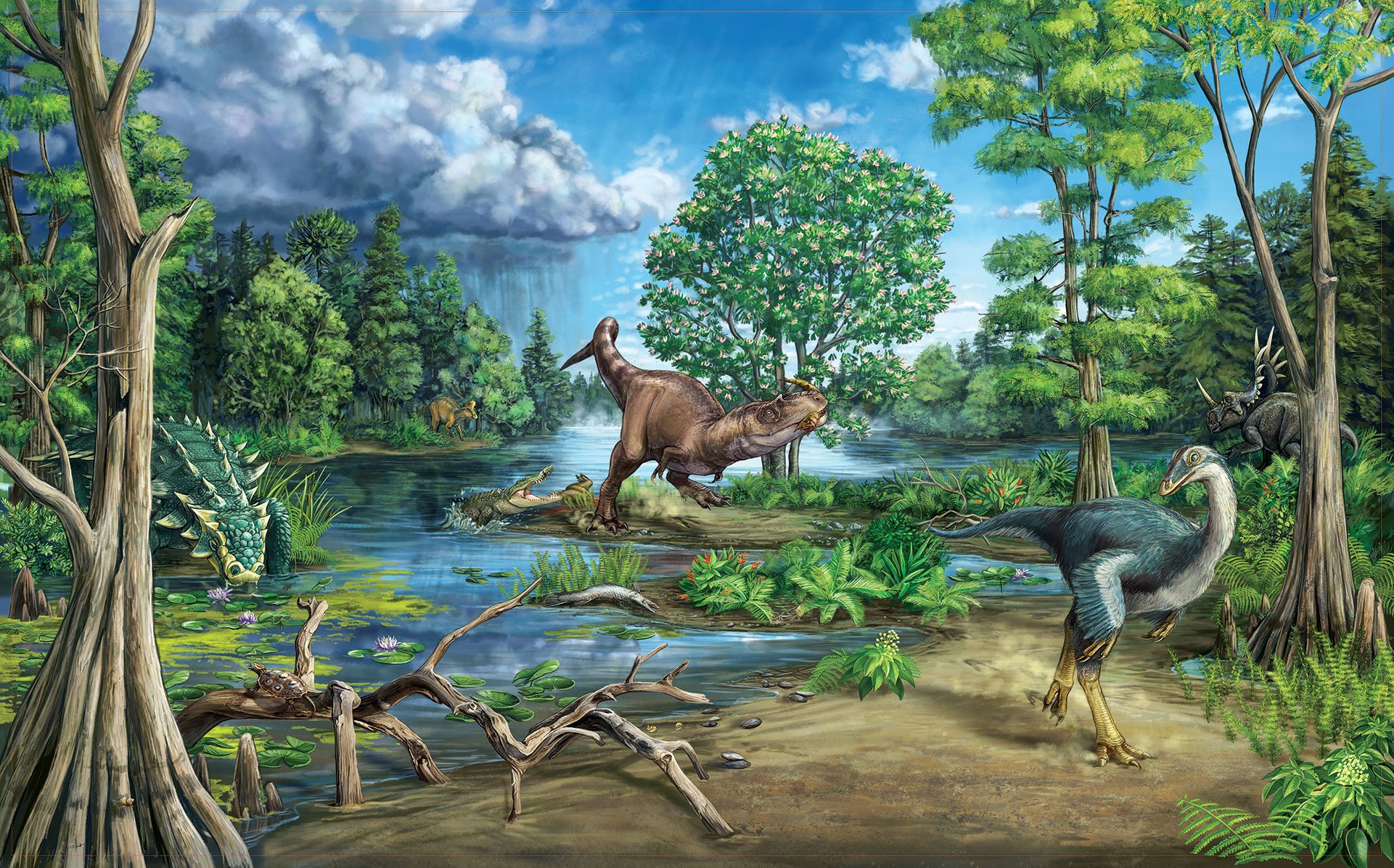The image is an intricate, detailed digital illustration or painting of a prehistoric landscape brimming with dinosaurs and lush vegetation. At the center of the scene, a brown Tyrannosaurus rex-like dinosaur charges towards the right. Nearby, a distinctive blue dinosaur with yellow legs coexists with other prehistoric creatures. To the right, partially obscured among dense foliage, a black dinosaur with a rhinoceros-like horn on its nose prowls. The foreground features dirt pathways and various plants, while the background reveals a serene waterway dotted with islands, each adorned with trees and greenery. A magnolia tree stands prominently behind the central T-Rex. Further in the background, a storm brews with rain already starting to fall, adding a dynamic atmospheric touch. The whole scene is rendered in a vivid color palette, rich in blues, greens, and browns, capturing fine details in both the natural elements and the dinosaurs themselves.